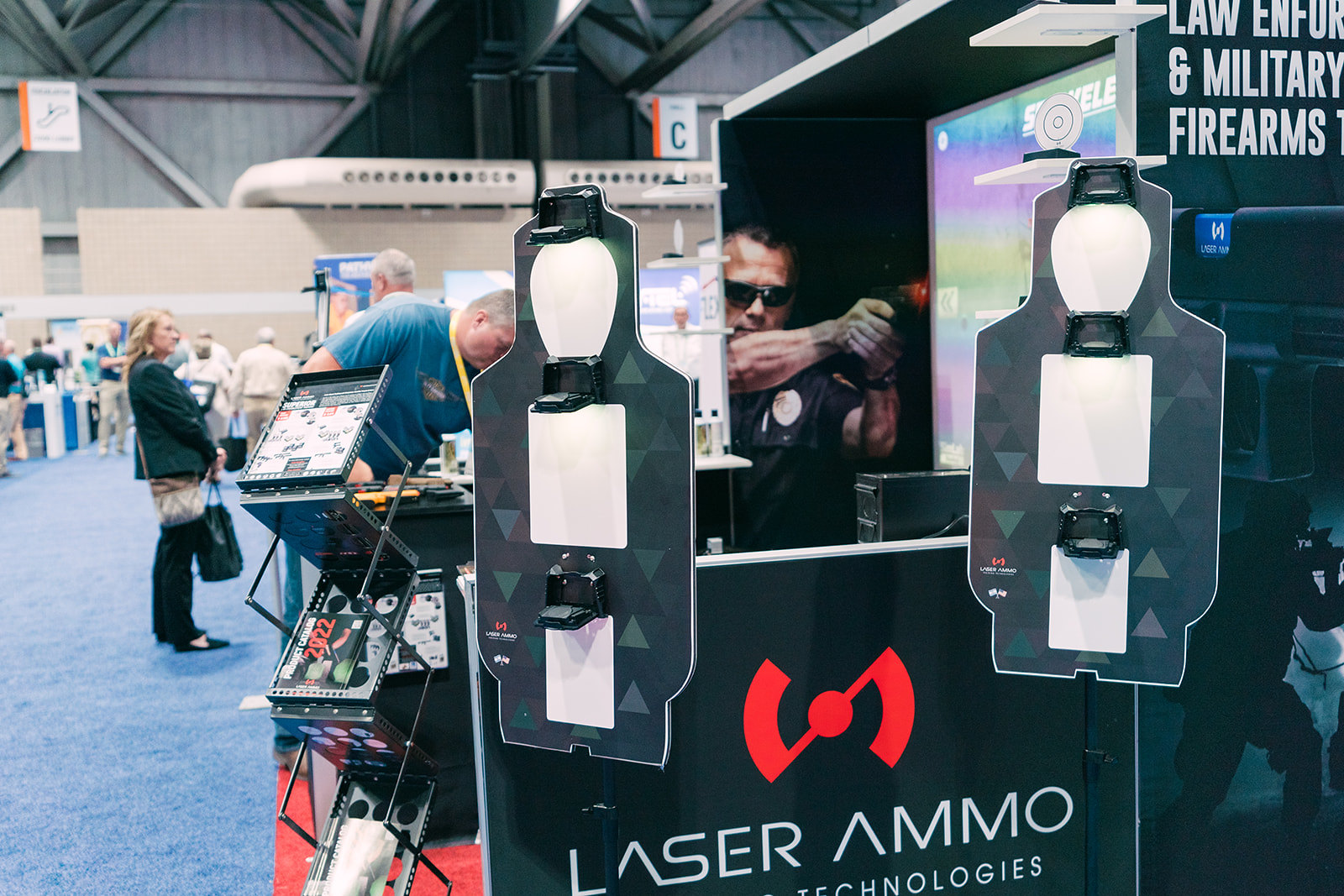The image captures a dynamic scene at a firearm trade show or convention, held inside a large convention center with blue carpeting and bright, overhead lighting. Prominently featured in the foreground is a man wearing dark shades, holding a firearm equipped with a laser sight. He is demonstrating this laser ammo technology to onlookers, aiming at two humanoid targets designed to mimic a head, torso, and waist, which are set against a camouflage backdrop. The booth, identified by a banner that reads "Laser Ammo Technologies," appears to be well-attended, with another man in the background wearing a yellow lanyard and leaning over to engage with the setup. To the left, a woman stands with her arms slightly outstretched, while beside her, a man with a yellow item around his neck bends forward. The booth also features a display screen with colorful patterns and a rack likely holding informational pamphlets or magazines related to the technology on showcase.